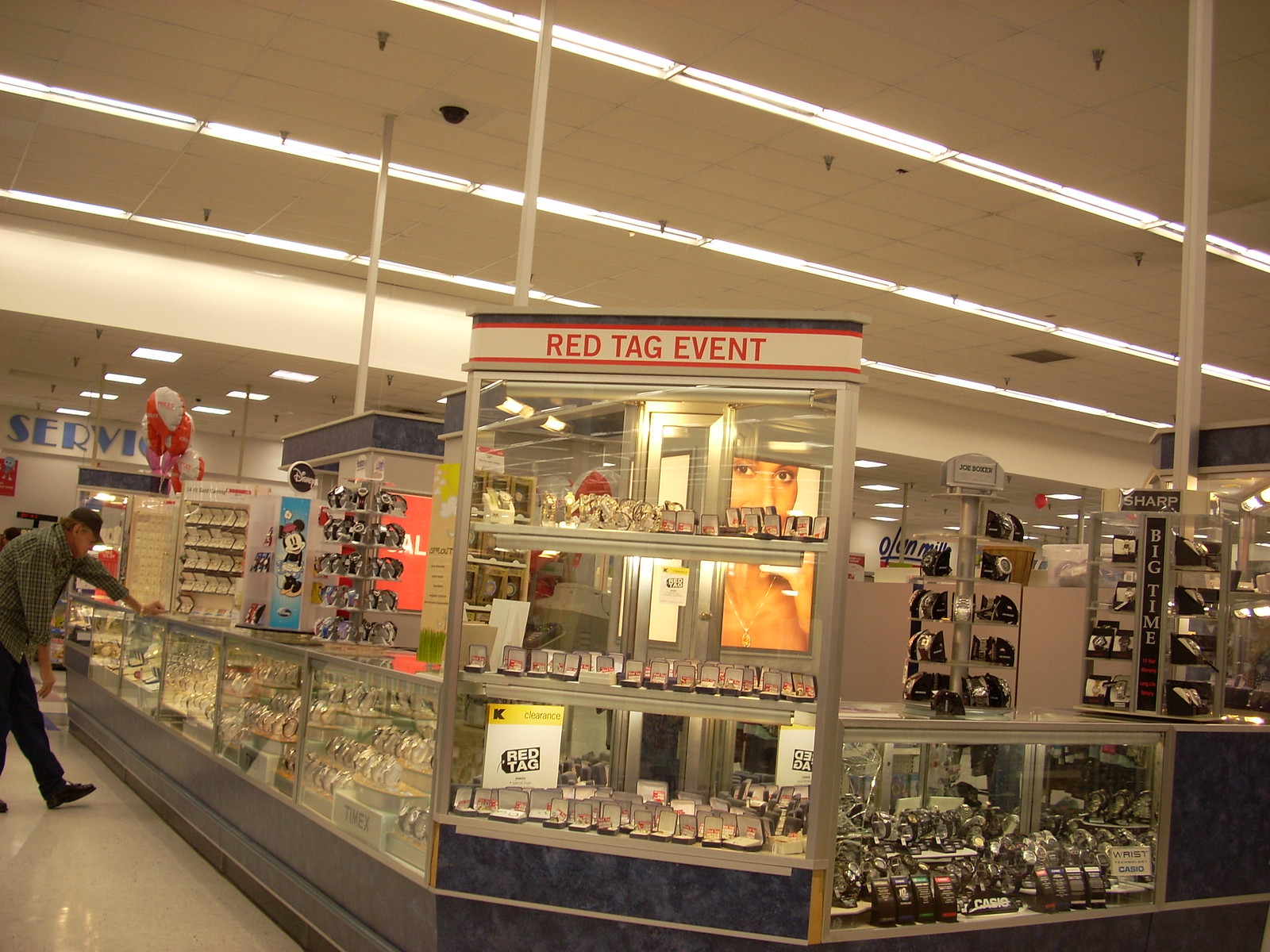This photograph captures a bustling scene at a department store's jewelry counter, offering a detailed view of a promotional event. The centerpiece is a three-layered shelf encased in glass, prominently featuring numerous open jewelry boxes with red tags indicating discounts, though the majority of the silver and gold jewelry remains partially hidden. Above this display, a white stripe with bold red text announces the "Red Tag Event," while a white sign with a yellow top and a black K logo beneath reads "Clearance." Inside the white section, a smaller black tag with white text reiterates the "Red Tag" theme.

To the right of the main display, a separate shelf showcases an array of watches, each neatly arranged and facing outward. Additional turntable shelves on the counter above also present more watches, creating an impressive array of timepieces. On the left side, a similar setup includes more watches on turntable shelves and additional shelving underneath, enhancing the comprehensive selection.

Standing to the left, a man dressed in a pale green, dark plaid shirt, dark pants, dark boots, and a dark hat leans against the counter, intently examining the items on display. His presence adds a human element to the scene, emphasizing the engaged shopping experience.